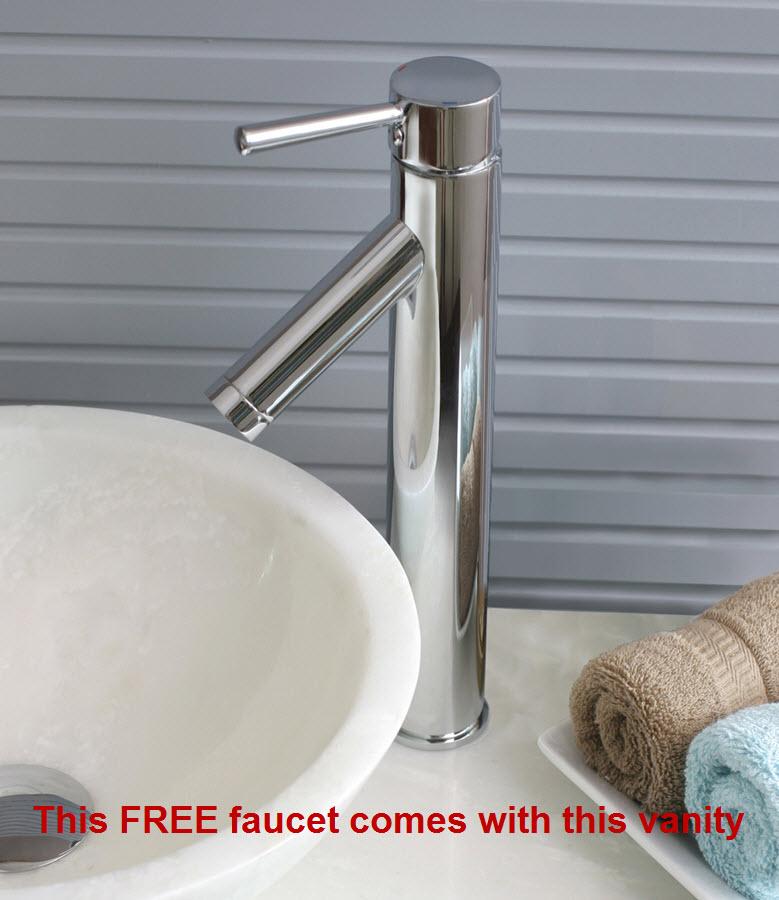This image appears to be part of an advertisement for plumbing fixtures, showcasing a modern bathroom setup. The central focus is a sleek, cylindrical, silver-colored faucet, which extends vertically from the bottom center to the top center of the image. It is situated on a white countertop that resembles formica or marble. Directly below the faucet is a circular white basin, with its drain visible in the bottom left of the image.

To the right of the faucet is a white tray holding two neatly rolled towels - the upper towel is brown and the lower one, partially obscured, is aqua blue. The backdrop is a gray wall featuring subtle vertical grooves or indentations, contributing to the contemporary aesthetic.

At the bottom of the image, across a red banner, the text reads, "This FREE faucet comes with this vanity," with "FREE" emphasized in all capital letters, highlighting the promotional offer.